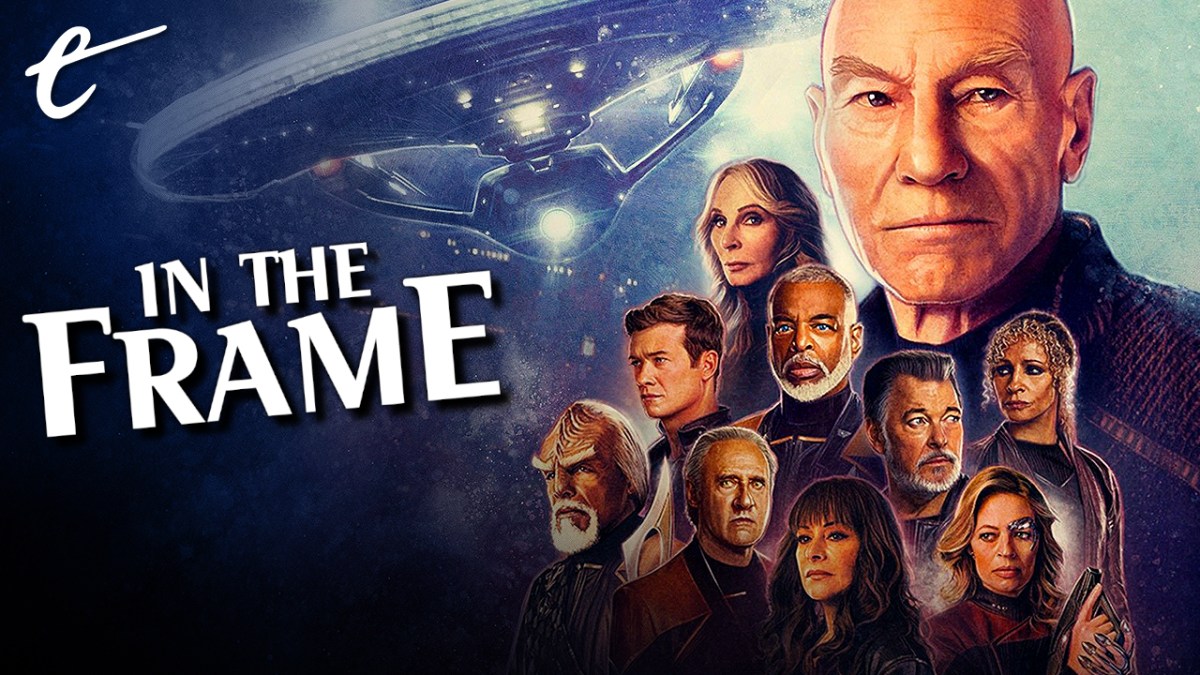This Star Trek poster features a striking photorealistic illustration reminiscent of Drew Struzan's style, showcasing the cast of "Star Trek: Picard." At the forefront is an enlarged depiction of Patrick Stewart as Captain Picard, his head and torso dominating the image, which conveys his central role. Surrounding him are nine other characters, including LeVar Burton, Jonathan Frakes, and Jerry Ryan, overlaid on his torso, depicting a cohesive ensemble cast.

On the top left and central part of the poster, a stylized spaceship, presumably the Starship Enterprise, traverses a dark blue sky. This spacecraft, identifiable by its distinctive shape and two bright lights, is truncated slightly by the frame. Above everything, a large cursive "T" along with a stylized "E," presumably symbolizing the Enterprise, is prominently featured.

The phrase "IN THE FRAME" appears in bold white capital letters on the left side of the image, with the words "in the" cleverly nestled between the taller "F" and "E" in "FRAME," creating a visually dynamic title. This vibrant assemblage of elements emphasizes the iconic Star Trek legacy while highlighting the specific "Picard" series.